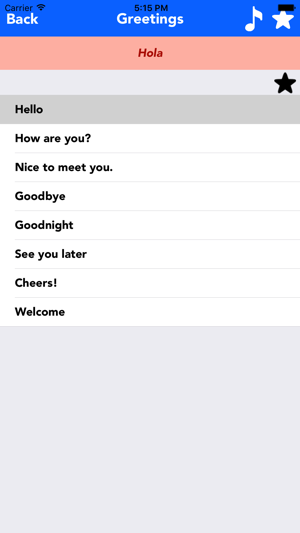The screenshot is vertically oriented and features multiple distinct sections. At the very top is a blue header with various elements. On the left side of the header, white bold text reads "Back". Centrally placed in the header is another set of white bold text that says "Greetings", which is flanked by a white music note icon and a white star icon. Just above the header, in the top left corner, is the word "Carrier" accompanied by a black WiFi icon. Adjacent to this, the time is shown as 5:15 PM, and a small battery icon indicates a full charge.

Below the blue header is a peach-colored banner with salmon-colored text that reads "Hola" or "Ola". Directly underneath is a gray banner featuring a black star icon positioned on the right side. Another gray banner follows, displaying the word "Hello" in black text. The next section is a white background with bold black text that reads "How are you?".

Each section is clearly delineated, making the visual hierarchy and various informational elements easily distinguishable.